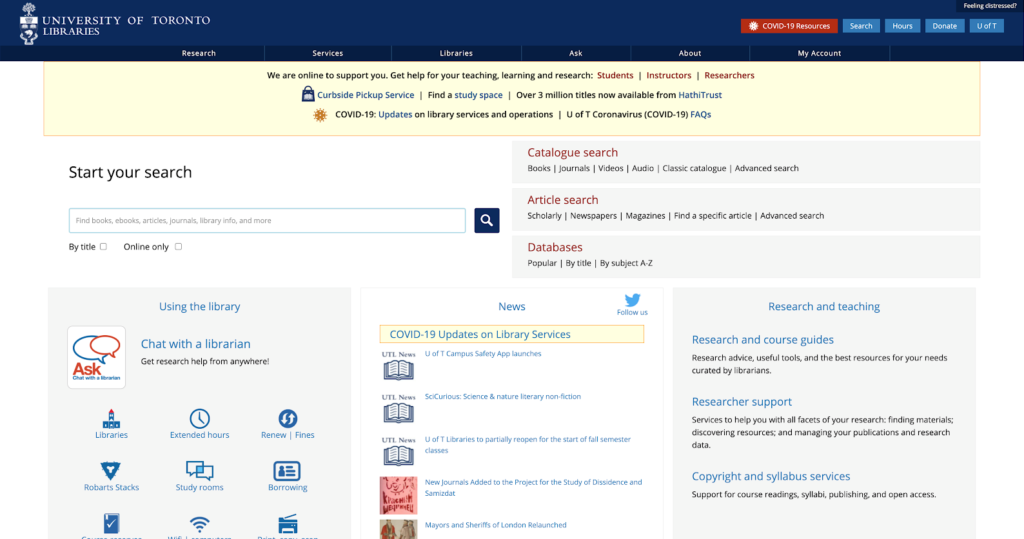A screenshot of the University of Toronto Libraries' webpage. Dominating the top part of the page is a dark blue rectangular banner, prominently displaying "University of Toronto Libraries" on the left side. The right side of the banner offers links to COVID-19 resources, search functions, library hours, donation information, research services, library locations, a question portal, an 'About' section, and account management. Below this banner, there is a notification that the librarians are online to assist, specifically providing help with teaching, learning, and research for students, instructors, and researchers.

Further down the page, users can access curbside pickup services, find study spaces, and view updates regarding COVID-19 at the University of Toronto. The middle section of the page provides various search options: catalog search, article search, and comprehensive database searches. Additionally, there is a prominent free-form search bar allowing users to enter any query directly. The page also features options to use the library services, chat with a librarian, or ask questions, all highlighted in light blue for easy navigation.